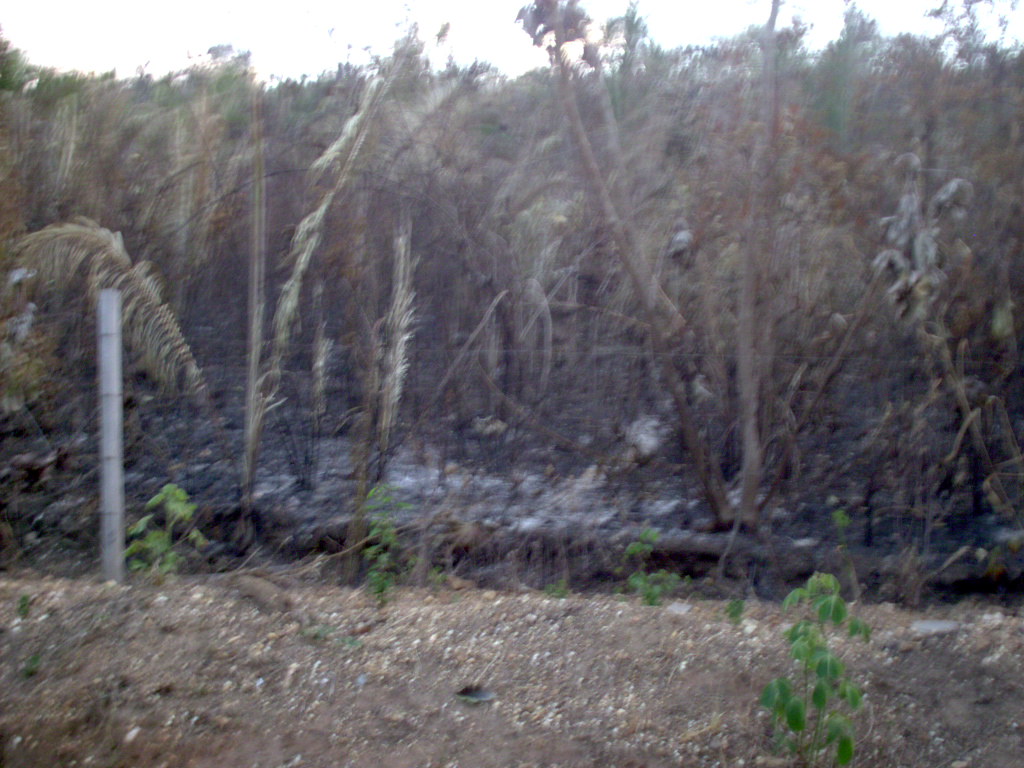This is a blurry photograph capturing a forest scene, possibly taken during winter or early spring before full bloom. The image is close-up, revealing brown trees that stand with a barbed wire fence in the foreground. A wooden post, grayish and about half the height of the trees, supports the barbed wire, with indications of a trench running alongside the fence. The ground is predominantly bare dirt with patches of dead grass and sparse white flowers, suggesting the season's dormancy. In the background, amidst an overcast, gray sky, are trees—some appear to be palm trees or fronds with bushy tops. The forest behind the fence exhibits signs of damage, with several trees lying on the ground, hinting at possible wind or fire destruction. The overall color of the photograph is muted, with a predominant grayscale tone, contributing to an eerie and somber atmosphere.